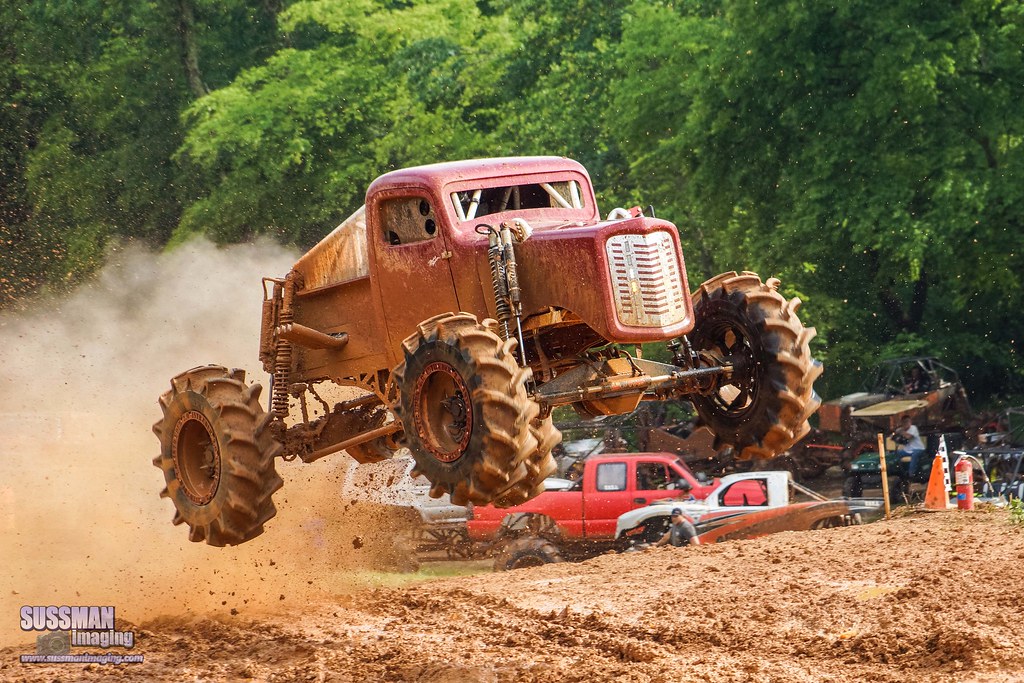In this outdoor image, a red monster truck with large, dirty wheels is captured mid-air, flinging dirt and dust behind it, indicative of an off-roading event or demolition derby. The photo also showcases a diverse background with several regular and monster trucks parked alongside, a man wearing a face cap beside a white truck, green-leaved trees, orange cones, and a fire hydrant. The bottom left corner features the text "Sussman Imaging" and "www.sussmanimaging.com" in white lettering.